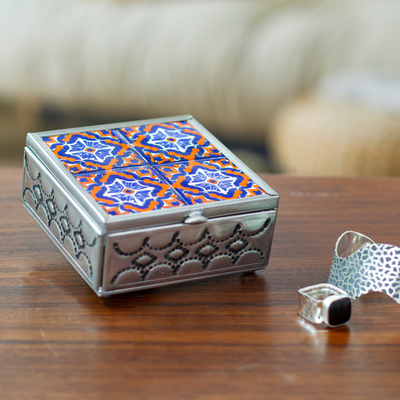This close-up photo captures a small, ornate silver trinket box, possibly a ring box, prominently displayed on a laminate wood grain table that shows light surface scratches. The background is intentionally blurred but hints at a gray object and maybe a sofa, ensuring all focus is on the intricately detailed box and the items beside it. 

The box is made of lightweight, light gray metal, featuring an ornate scalloping design along the top and bottom edges, with small diamond-like embellishments in between. The box’s lid showcases a stunning arabesque mosaic tile design divided into four quadrants, each featuring medium blue, orange, and white patterns that resemble star or floral motifs. 

Positioned slightly tilted to the back, the box has a clasp mechanism at the front, suggesting it can be opened. To the right of the box on the table are two pieces of jewelry: a textured, chunky silver ring with a large black gemstone and another smaller silver ring or circular object, possibly an art piece, adding to the sophisticated arrangement. 

The craftsmanship and design elements of both the box and the jewelry suggest a high level of detail and care was taken in creating this visually appealing scene.